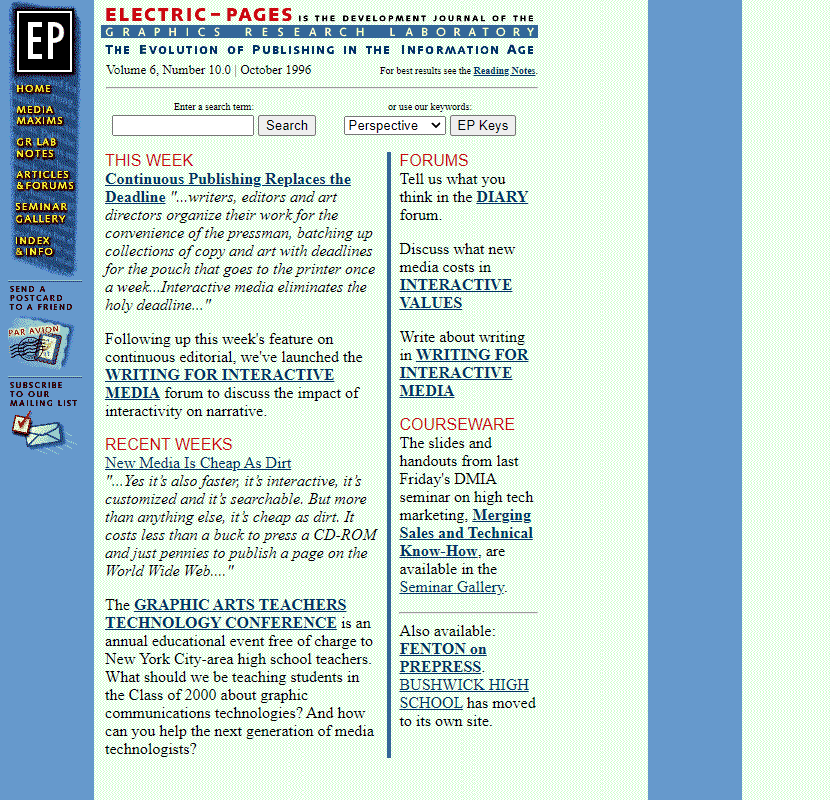This image showcases a website titled "EP" enclosed within a dark black square with a white outline. The acronym "EP," written in white, stands for "Electric Pages." This website serves as the development journal of the Graphics Research Laboratory, documenting the evolution of publishing in the Information Age. The edition featured is Volume 6, Number 10 from October 1996.

A reading note is recommended for optimal navigation. Users can enter search terms or use keywords to browse the site. The webpage highlights that continuous publishing has replaced traditional deadlines, focusing on writing for interactive media and its values.

The site encourages user interaction, inviting visitors to share their opinions in diary form. Additionally, it offers courseware, including slides and handouts from a recent high-tech marketing seminar held the previous Friday.

The layout is divided into two vertical sections, with information running down the left and right sides. Two vertical blue lines demarcate these sections. 

The left sidebar features links labeled "Home," "Media Maxims," "GR Lab Notes," "Articles and Forums," "Seminar Gallery," "Index," and "Info." It also provides options to send a postcard to a friend and subscribe to a mailing list, emphasizing the site's comprehensive and information-rich nature.